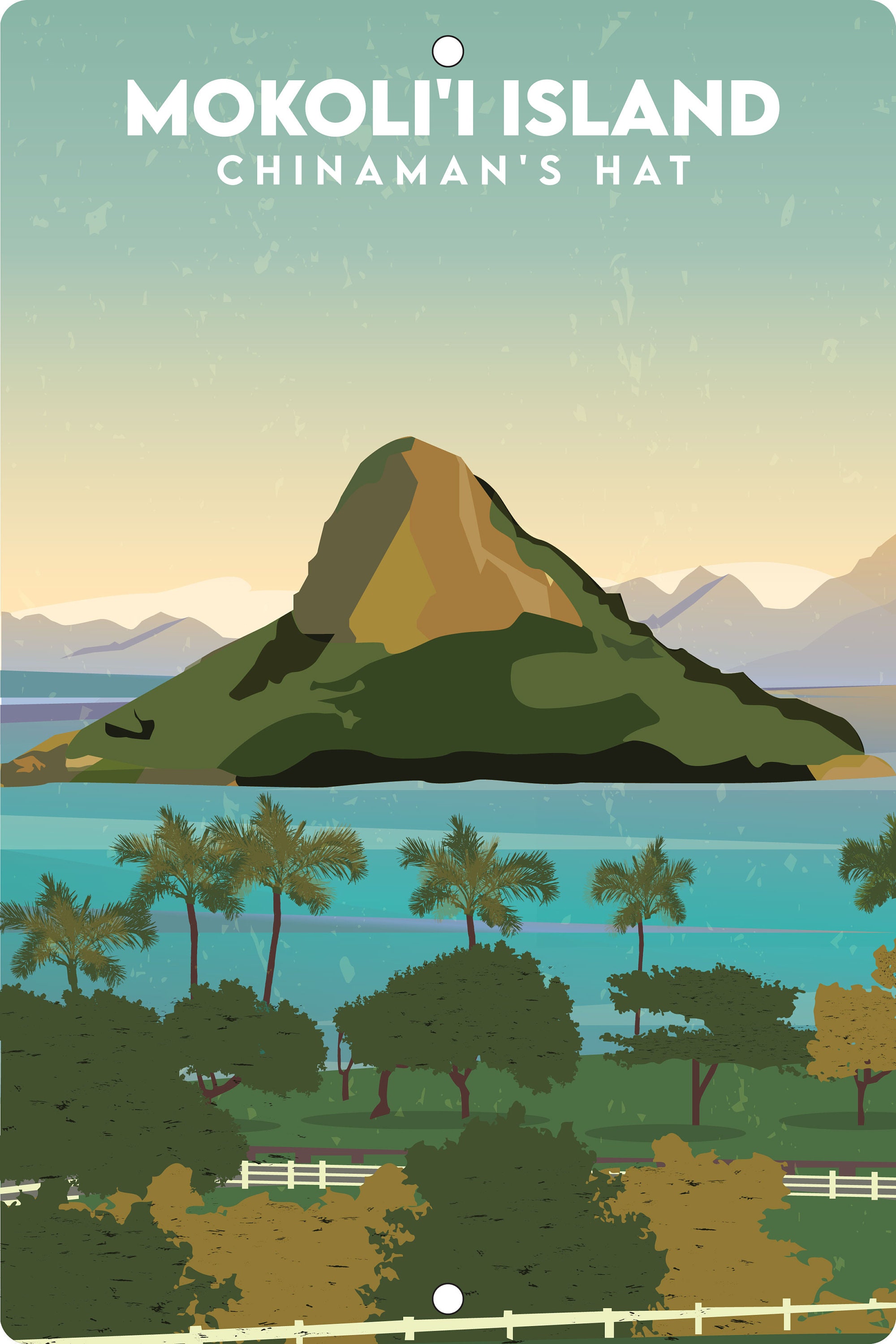This vertical rectangular poster features a digitally created landscape illustration advertising Mokoli'i Island, commonly known as Chinaman's Hat. Dominating the upper portion of the image, bold white capital letters announce "Mokoli'i Island" with "Chinaman's Hat" written beneath in smaller text. Above this lettering is a prominent white circle. At the center of the poster, the island itself is depicted, resembling a traditional Chinaman’s Hat and sitting loftily upon the water. The middle of the image showcases this hat-like natural rock formation, with distant gray-tinged mountains extending into the background, some displaying subtle purple hues.

Towards the bottom fourth of the poster, the scene transitions to the shore, populated with lush green trees, palm trees, and fencing that winds horizontally across the landscape. The foreground includes a vibrant blend of colors: greens, tans, golds, along with patches of blue and gray, reflecting the surrounding water and sky. The entire composition is framed within a serene sky backdrop, which completes the picturesque and inviting portrayal of Mokoli'i Island, emphasizing its unique geological feature and tropical environment.